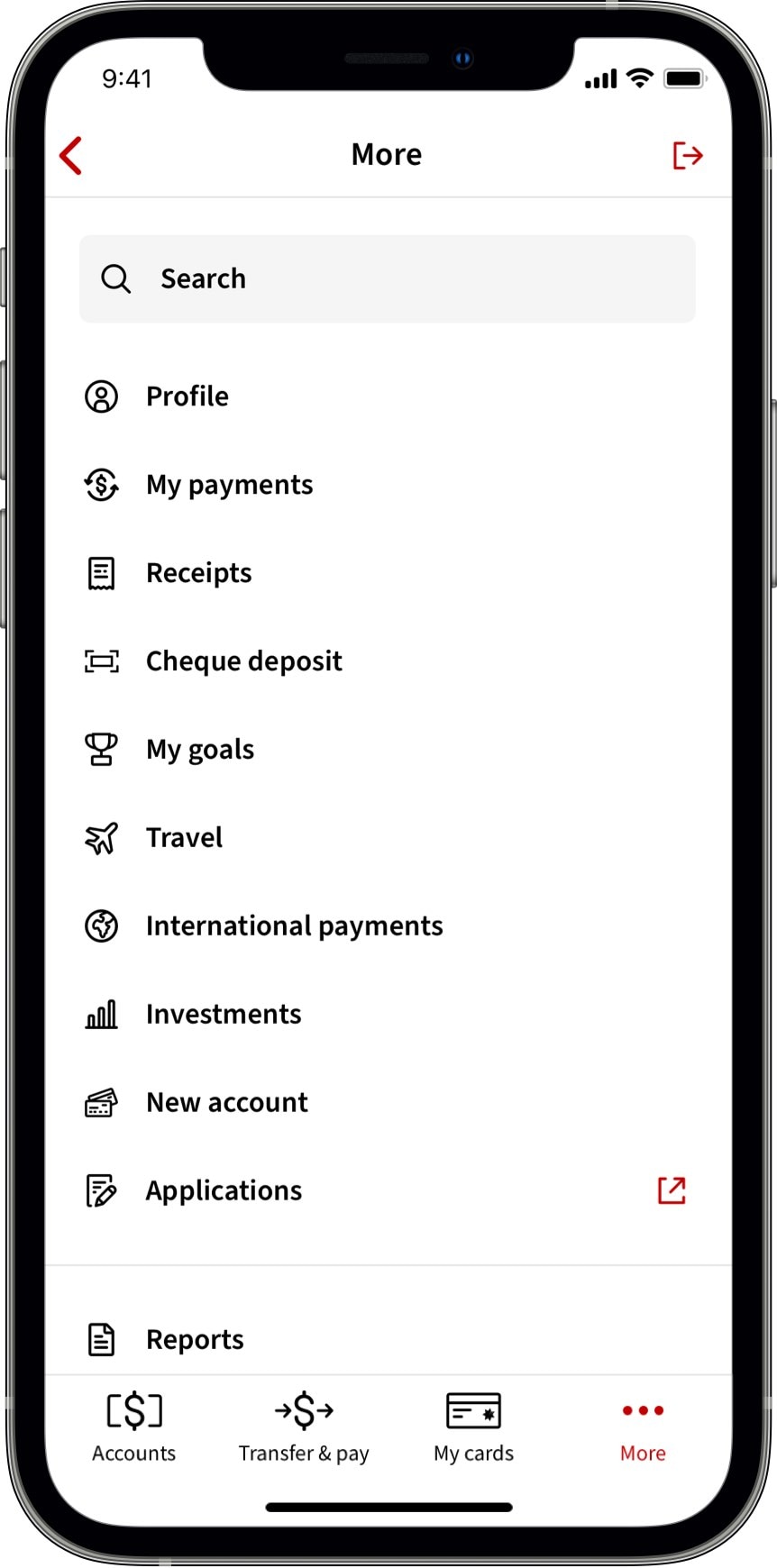A screenshot captures an entire physical smartphone along with its displayed content. The phone, featuring a silver volume button on the right side and three buttons on the left (including the power button), showcases its interface at 9:41 AM. The display is on a "More" page within what appears to be a money management application. The phone has two front-facing cameras positioned at the top and it shows full Wi-Fi signal, full cellular bars, and a fully charged battery.

On the app's screen, the top navigation includes a back arrow and a forward arrow, flanking the "Morris" section, accompanied by a search box labeled "search." Below this are menu options: Profile, My Payments, Receipts, Check Deposit, My Goals, Travel, International Payments, Investments, New Accounts, and Applications (highlighted with a red upward arrow). At the bottom of the screen, a section labeled "Reports" is accompanied by four navigation buttons: Accounts, Transfer and Pay, My Cards, and More, each enhanced with a corresponding icon and three red dots indicating notifications.

Each menu option is identifiable by a unique icon—for instance, a person silhouette for Profile, a money symbol circled for My Payments, a trophy for My Goals, and an airplane for Travel. This detailed screenshot provides a comprehensive look at the functionalities offered by the financial management app.